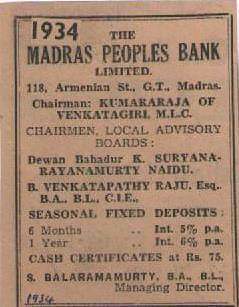A worn, peach-colored piece of paper, possibly a newspaper cutout, features black printed text with a border framing the content. The document prominently displays "1934" in bold, followed by "The Madras People's Bank Limited" at "118 Armenian Street, G.T. Madras." Several authoritative names are listed: the Chairman, Kumara Raja of Venkatagiri, MLC; the Chairman of Local Advisory Boards, Dewan Bahadur K. Suryanarayanamurti; and B. Venkatapathy Raju, Esq, B.A., B.L., C.L.E. It also details financial offerings, including "Seasonal Fixed Deposits" with six-month interest at 5% and one-year interest at 6%, alongside "Cash Certificates at Rs. 75." The Managing Director is noted as S. Balaramadurti, B.A., B.L.